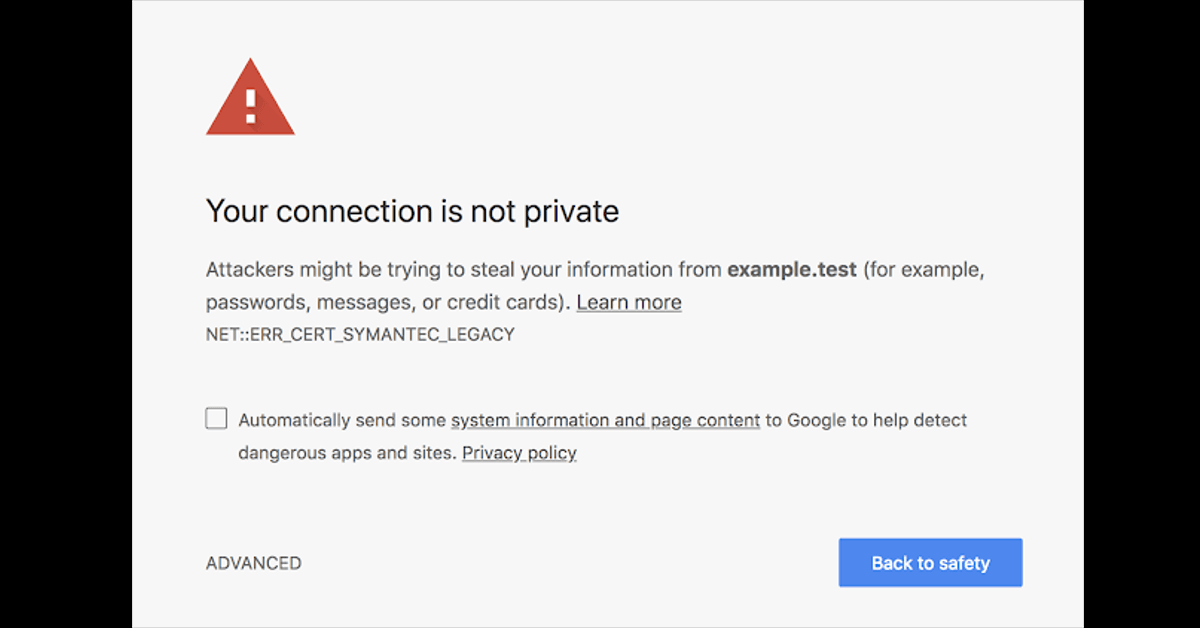"An image showcasing a security warning screen with a prominent message indicating 'Your connection is not private' in bold black text at the center. Above this warning, a red triangle with an exclamation point serves as an alert symbol. Directly below, the message continues: 'Attackers might be trying to steal your information from example.test (for example, passwords, messages, or credit cards).' To the right of this warning, 'Learn more' is underlined, offering additional information. At the bottom, there is a technical error code in all caps: 'NET::ERR_CERT_SEMANTIC_LEGACY'. Additionally, a checkbox option labeled 'Automatically send some system information and page content to Google to help detect dangerous apps and sites' is present but not selected. Near the bottom of the screen, there are two options: 'Advanced' on the left and 'Access Safely' in a blue hyperlink box on the right. The sides of the screen are framed by black borders, resembling a blackboard effect."